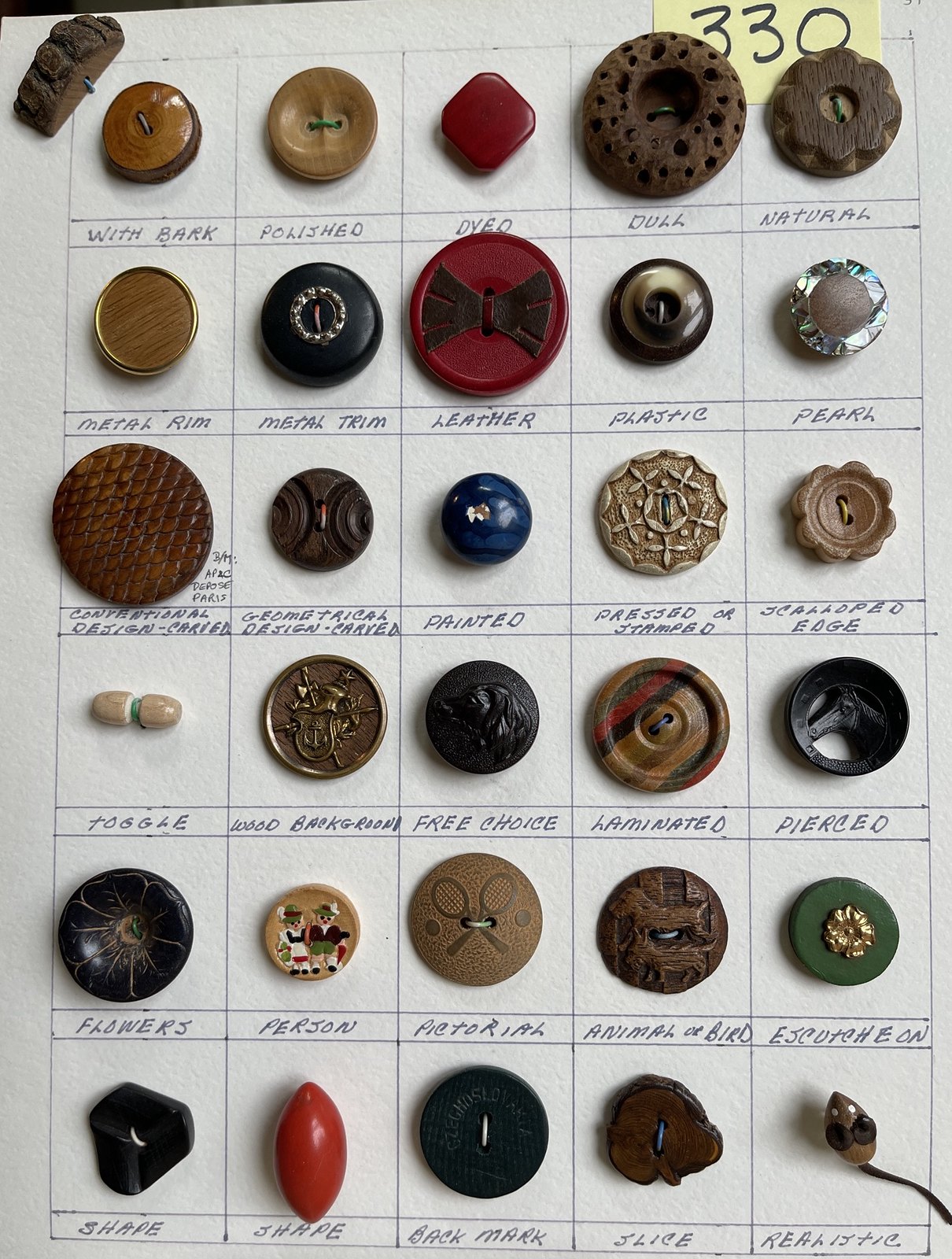This image showcases an intricate collection of antique and decorative buttons meticulously arranged on textured white paper. The buttons are displayed in a grid layout, each placed within a tile and accompanied by hand-written descriptions on tags underneath. The top-left tile features a circular wooden button labeled "with bark," followed by a polished button that resembles a wine bottle top. The second row includes a red-dyed leather button in the middle and pearl buttons on the right, while other buttons are more ornate in design. Notably, the third row has a standout blue button among mostly brown decorative buttons. There are specific buttons that catch the eye: a brown wooden button with a flower shape, a button depicting tennis rackets, a smooth button with a central dimple, and a red button with a brown leather bowtie. The fourth row contains black buttons with unique designs, and the fifth row features buttons with little German figures. One row also has a button with a mouse shape, adding to the unique and diverse collection. Various other detailed buttons include a green round button with a golden flower, a pill-shaped shiny red button, and a donut-shaped button. Lastly, the labels describing them use various terms such as polished, dyed, dull, plastic, pearl, painted, free choice, and pierced, offering a detailed insight into the diverse artistry and design of the buttons.